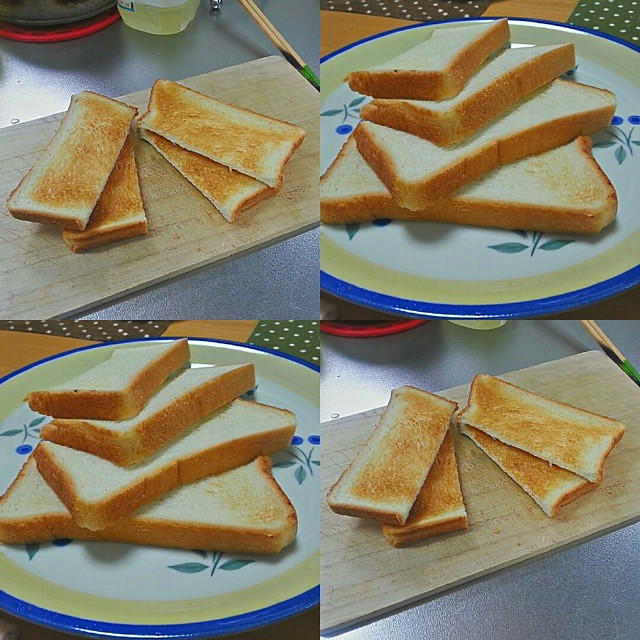This composite image features four photographs of different toast arrangements, meticulously laid out to emphasize symmetry and subtle variations. The upper left and bottom right images capture four medium-toasted half slices of bread, arranged fan-like on a rustic, rectangular wooden cutting board sitting atop a grayish blue countertop. Accompanying them are small background elements like bottles and a tiny cup with yellow juice. The upper right and bottom left images display four slightly toasted slices of bread, some whole and some halved, stacked in a cascading pile on an elegantly designed white plate. These plates feature intricate floral patterns with blue flowers, a golden ring, and a blue border, adding a touch of vintage charm. The plates rest on a wooden table with green and white polka-dotted placemats. Though the toasts in each quadrant differ slightly in their arrangements, the mirrored layout ties the composition together.